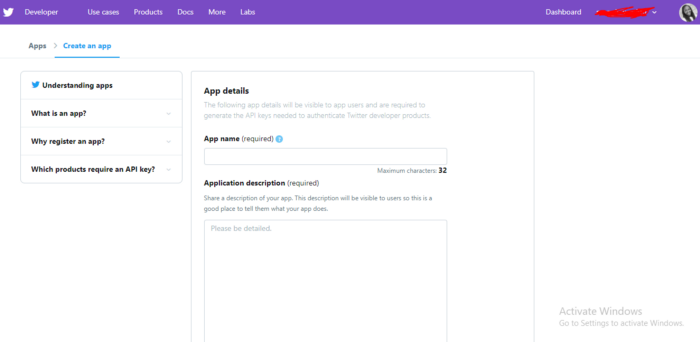This is a detailed screenshot of a website, showcasing its user interface elements. At the top, there is a purple navigation bar with several menu options in white text: starting from the left, the options are "Developer," "Use Cases," "Products," "DOCS," "More," and "Labs." On the right side of this bar, the navigation options include "Dashboard," followed by a vertical red slash, and a circular icon containing a person's profile image.

Below this navigation bar, the layout is organized into two main sections. On the left side, there is a white background with the heading "Apps." An arrow points right to the blue, underlined text "Create an App." Beneath this, a grey-outlined box contains four items of data: 
1. "Understanding Apps"
2. "What is an App"
3. "Why Register an App"
4. "Which Products Require an API Key"

The center section features a larger grey-outlined box titled "App Details." It explains that the details provided here will be visible to app users and are necessary to generate API keys for authenticating Twitter developer products. Within this section, there are fields labeled "App Name (required)" with a text box for input, followed by a note, "Maximum characters: 32." Below this, there is another text box labeled "Application Description."

Finally, in the bottom-right corner of the screenshot, there is a watermark that reads, "Activate Windows," with an instruction to "Go to Settings to activate Windows."